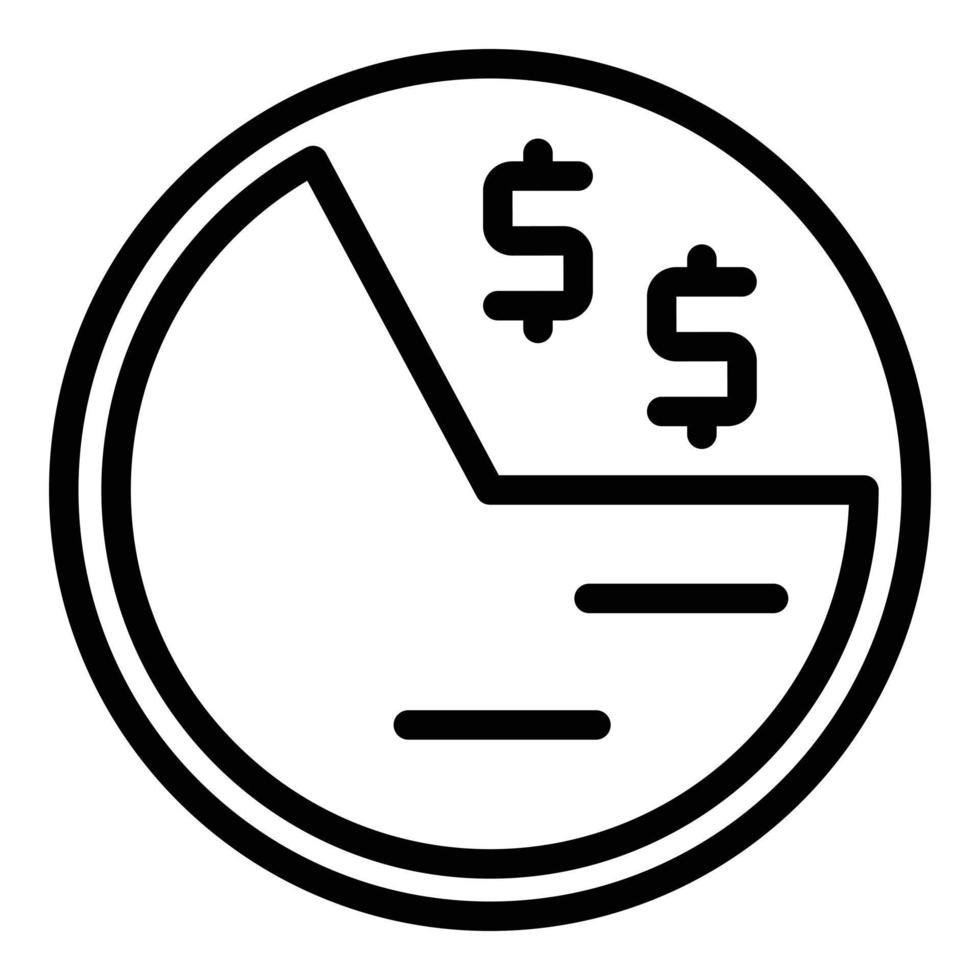The artwork is a square-shaped image framed by a small white border. Dominating the piece is a large circle with a thick black outline and a white interior. Towards the bottom left of this circle, a wedge-shaped section, akin to a Pac-Man shape, is removed, ranging from approximately 11:30 to 3 o'clock. Within this wedge area, two vertical black lines are visible near its center. Above this cut-out section, near the upper right side of the large circle, there are two distinct dollar signs, each characterized by an "S" shape with two horizontal strokes at the top and bottom. The entire composition is rendered in stark black and white, emphasizing the contrasting geometric forms and symbols within the piece.